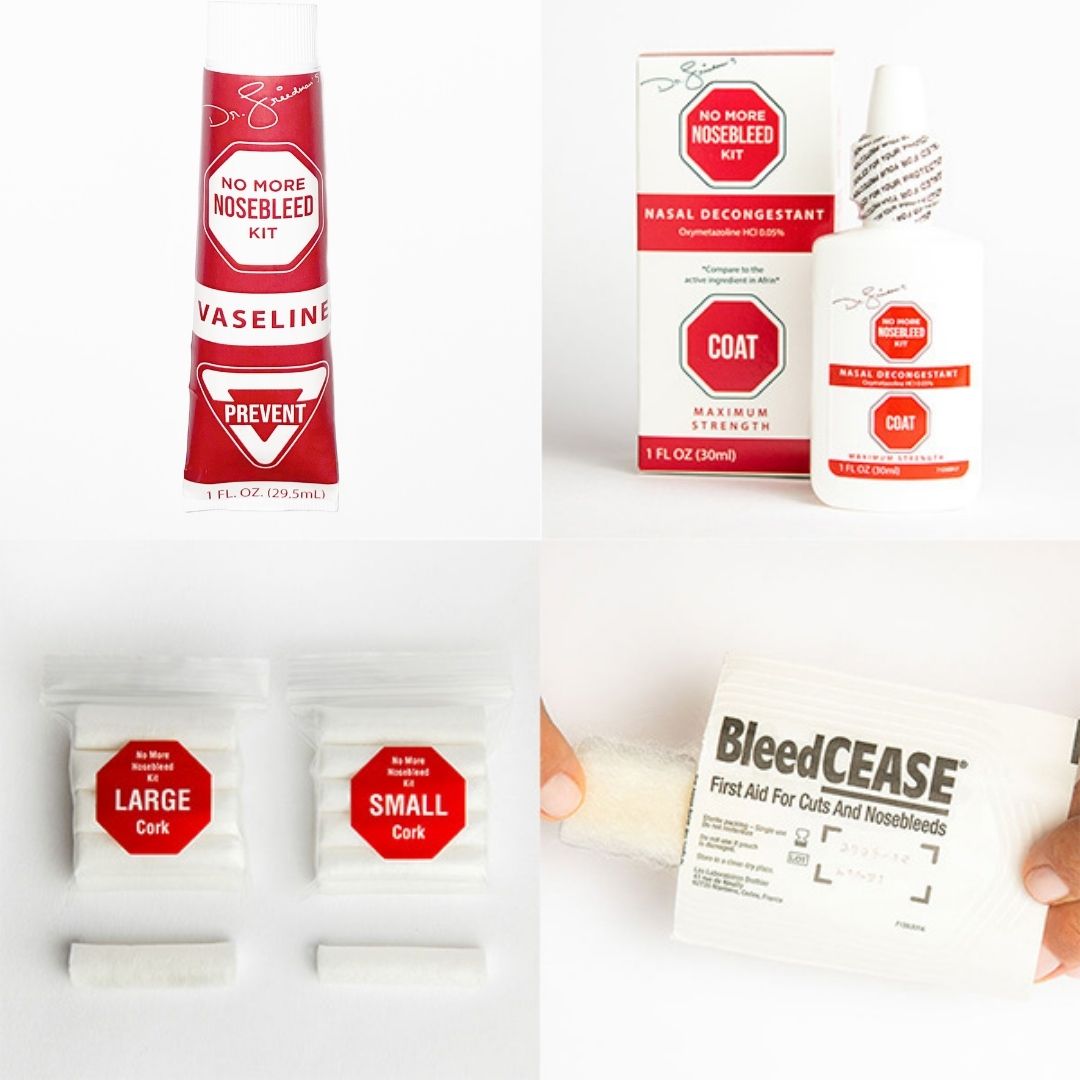The image is a photographic composition of four distinct shots of first aid items tailored for nosebleed prevention and treatment, likely set indoors. 

In the top left, a red and white tube labeled "No More Nosebleed Kit Vaseline Prevent" is prominently featured. This tube, designed to prevent nosebleeds, includes clear text in black and white.

Adjacent to this, on the top right, is a packaging display for a nasal decongestant. The package includes both a box and a bottle labeled "No More Nosebleed Kit, Coat, Nasal Decongestant, Maximum Strength, One Fluid Ounce, 30 mLs." The text above "COAT" and part of the nasal decongestant's formula name, "Oxy-something HO" alongside a small percentage, are present but difficult to read. Both the box and the spray bottle share the same red and white color scheme and textual details.

On the bottom left, there are two plastic bags containing white corks meant to stop nosebleeds. One bag houses a large cork, and the other a small cork, both marked with red text reading "No More Nosebleed, Large Cork" and "No More Nosebleed, Small Cork," respectively.

The bottom right showcases a close-up of a woman’s fingers holding a white package labeled "BLEED CEASE, first aid for cuts and nosebleeds," printed in black lettering. The word "CEASE" is both capitalized and underlined. The background of the packaging is white, and there is additional, though unreadable, text in gray on the back.